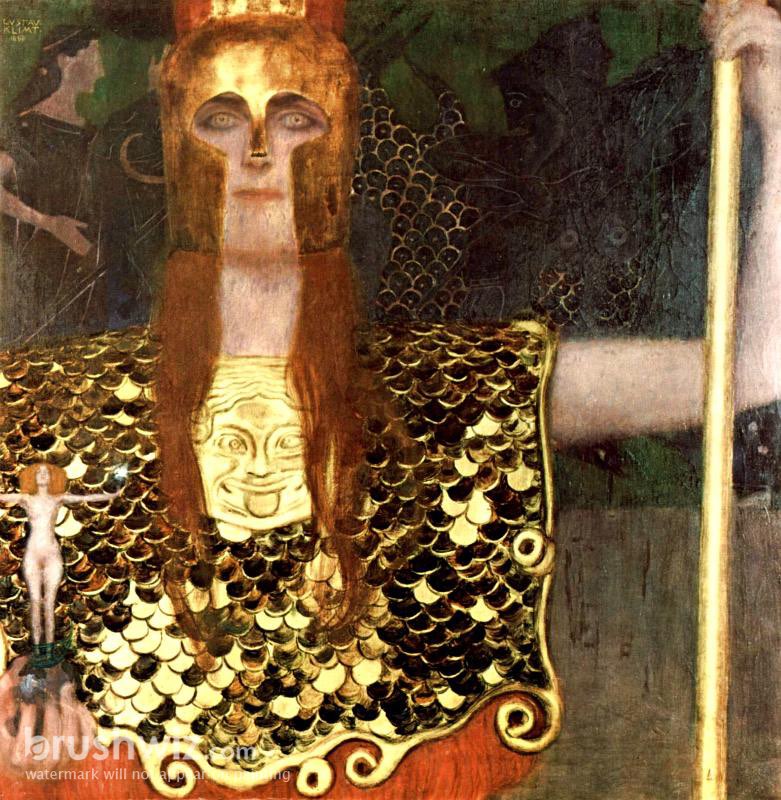The image is a detailed painting featuring a prominent woman with long, red hair and pale skin, looking directly at the viewer. She is adorned in gold chain armor, with a gold-plated vest resembling scales, and a face on the chestplate sticking out its tongue. She wears an ancient Greek or Roman style golden war helmet and holds a gold staff in her left hand. In her right hand, she holds a small statue of a naked woman with red hair, depicted in a T-pose with arms outstretched. The background includes various elements: a robed figure with dark hair, another person in green colors, and a monstrous creature with huge eyes and a human-like face. On the left side of the image, there's a visible watermark reading "Broomswiz.com" with additional indistinct text.